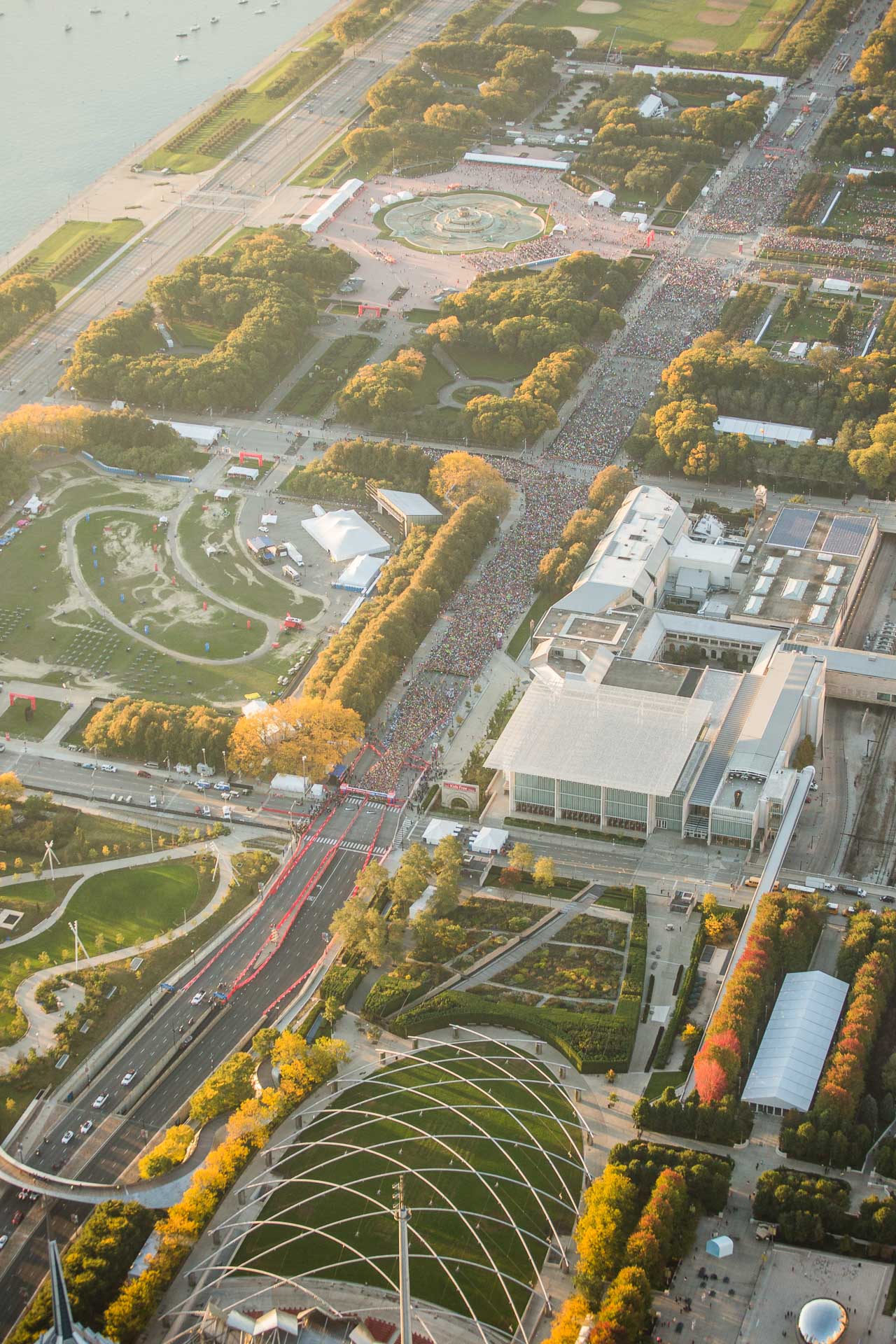This aerial shot, likely taken by a drone, reveals a meticulously planned cityscape, blending urban development with abundant greenery. Dominating the image is a wide, six-lane road that diagonally stretches from the upper right to the lower left, appearing to host a vibrant parade with people gathered in the center. Surrounding this main road, the city layout is divided into squared sections of land.

To the bottom right, a lush green field is juxtaposed with a large white building complex above it. Further up, dense clusters of vibrant yellow-leaved trees add a striking contrast. On the left side of the road, a sprawling park features an outdoor amphitheater nestled among more green spaces. Additionally, the upper left corner of the image unveils a scenic harbor with sparkling water.

Intriguingly, a silver wire-like structure covers the top part of the image, forming a dome that encompasses the scene. It’s clear that despite the urban elements, the city maintains a balance with nature through its numerous parks and tree-lined areas.